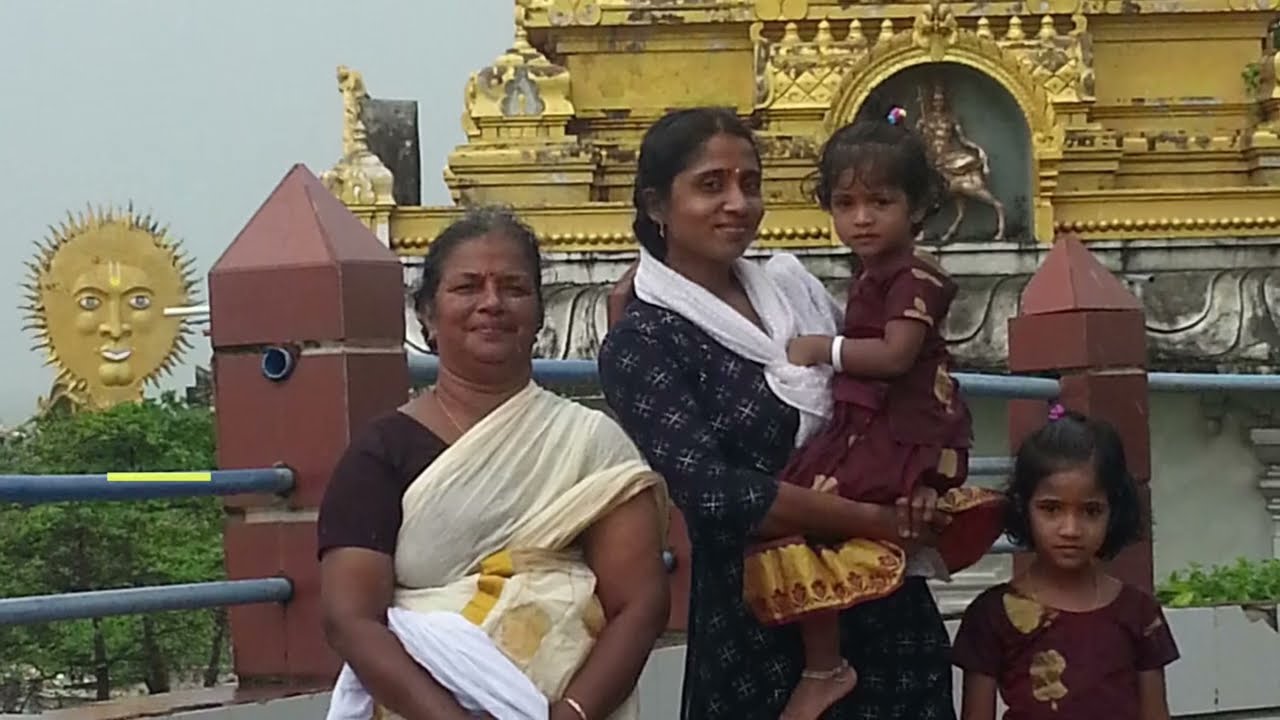The image portrays a multi-generational Middle Eastern or South Asian family, possibly of Indian or Pakistani descent, posing joyfully for the camera in front of an ornate golden temple. The family consists of a grandmother, a mother, and two young daughters, signifying three generations. The backdrop features an elaborate temple with golden decorations and statues, including a notable statue of a sun with a face and another statue resembling a horse or a centaur. The temple rests on a medium gray stone base, and the family is positioned behind protective maroon posts with metal bars.

In the foreground, the grandmother stands on the left, donning traditional attire that includes a white sash. The mother, positioned beside her, is dressed in a dark-colored dress with a star pattern, complemented by a white sash. The two daughters stand to the right, both dressed in matching maroon and gold dresses with gold bracelets adorning their wrists and ankles. They are all smiling warmly, capturing a happy family moment against the stunning backdrop. The scene suggests they are on a deck-like area, indicated by the horizontal beams acting as a safety fence, with hints of greenery and an elevated vantage point behind them.